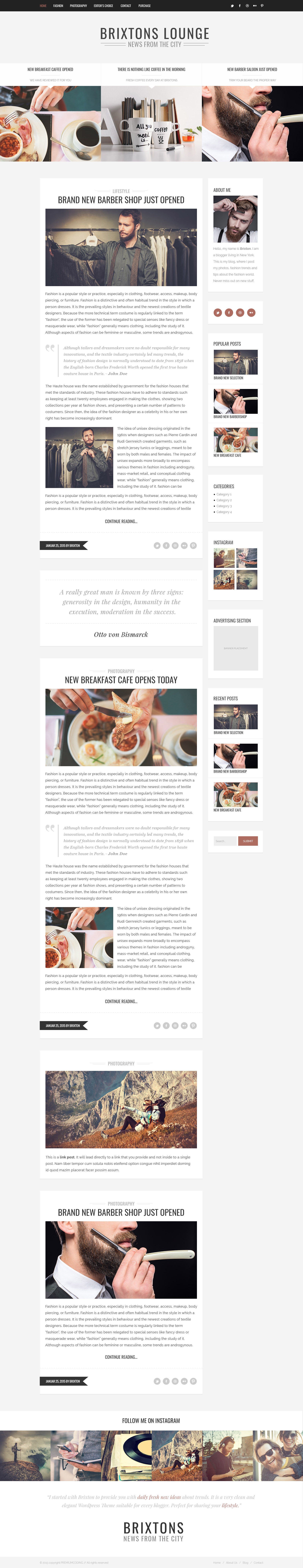The web page for Brixton's Lounge is quite cluttered, featuring numerous images and extensive text in an exceedingly small font, making it difficult to read. At the top of the page, prominently displayed in a rectangular slot, is a banner image showcasing food and drink. The images throughout the page appear disorganized and are presented at awkward angles, further obscuring their clarity. The top banner includes a scene with a man standing before a waterfall, while the intervening images predominantly display various dishes. Among these, there is also a picture of a shingly beach. At the bottom of the page, an image depicts a bearded man holding an object up to his face, though the object is difficult to identify. It remains unclear whether Brixton's Lounge is a restaurant or a hotel, but the focus seems to be on food, drink, and some scenic views.